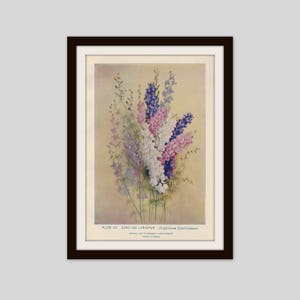In the image, we see a framed piece of art, possibly a photograph of a painting or print, featuring an array of vibrant flowers set against a background that appears to be discolored parchment. These flowers, which may be snapdragons or foxtail-like in form, display a range of colors including white, pink, purple, blue, and green. The flowers are densely packed and arranged in a vertical manner along their stems, creating a visually pleasing bouquet that resembles the shape of a corn on the cob. Below the arrangement, there is some small, illegible text. The artwork is mounted in a black wooden frame with at least one matte, and the entire piece is displayed against a white background, which appears gray in the photograph due to lighting. The setting is starkly simple, with no additional elements in the image.